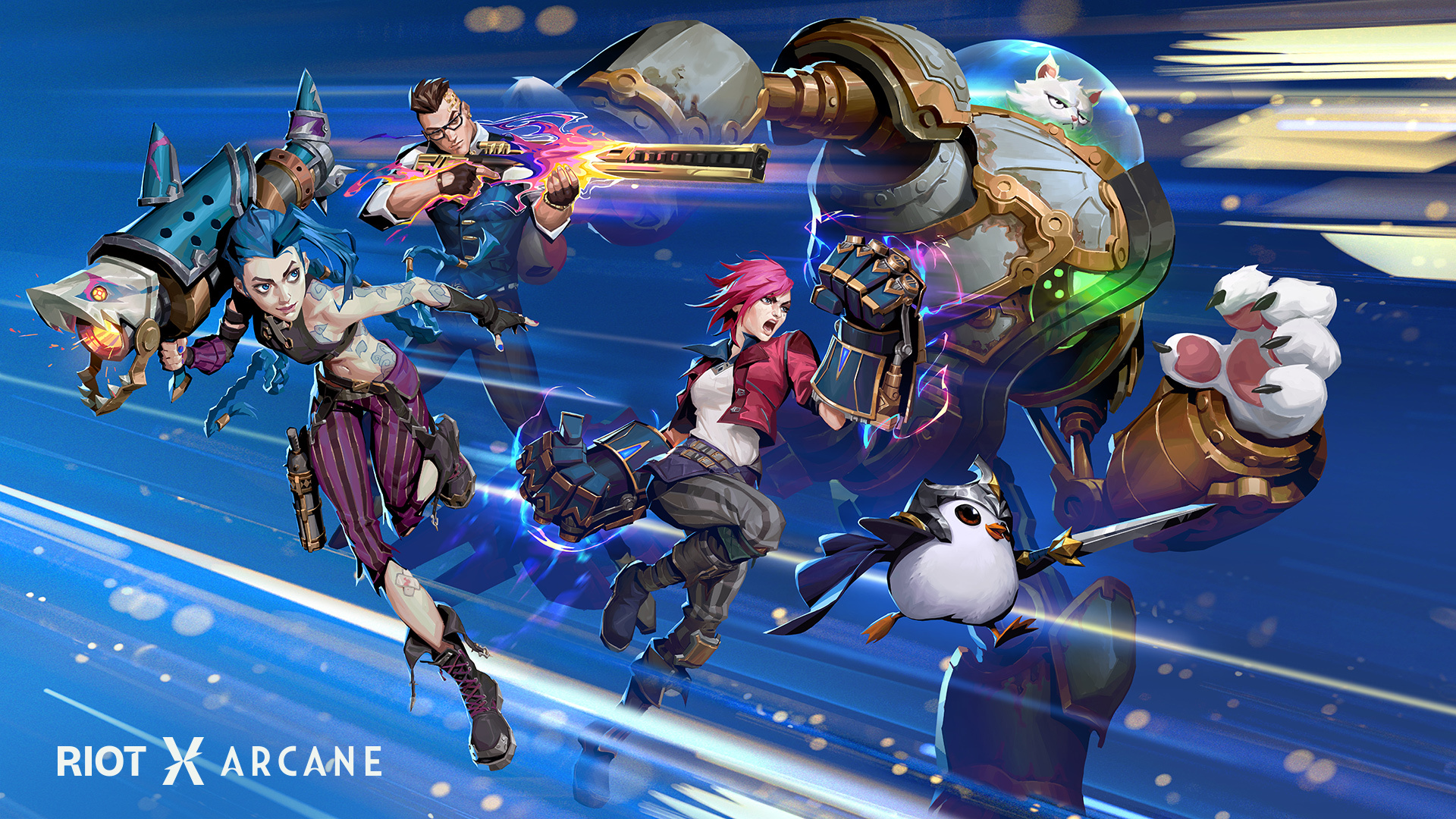The image is a dynamic digital graphic, seemingly an illustration for a game or cartoon titled "Riot X Arcane," as indicated by the white lettering in the bottom left corner. Set against an intense blue background streaked with white lines to depict high-speed action, the scene teems with vibrant characters in mid-motion. Central to the composition is an oversized robotic figure with a turret where its head should be and a massive barrel gun jutting out. To its left stands a muscular soldier clad in a blue uniform, crew-cut hair and glasses, brandishing an elongated gold rifle. The scene also features two women flying or swimming through the sky, dressed in halter tops and purple and black capri pants with black boots. Additionally, there's a whimsical penguin wielding a sword with determination, and a figure in a cat-like robotic costume equipped with a glass shield. The characters, each exuding a unique flair with their vividly colored appearances, appear to be in a combat or chase sequence, adding to the image's overall sense of frenetic energy.